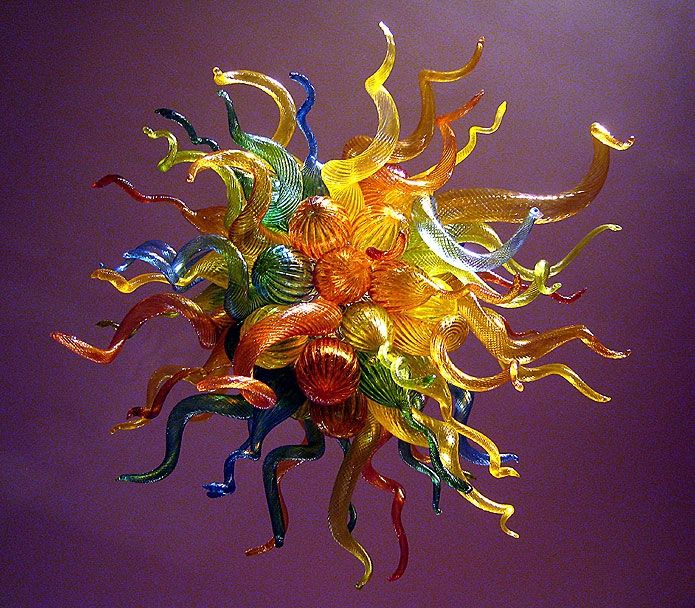The artwork is an abstract, multicolored blown glass sculpture set against a dark magenta or purple background. The piece features numerous swirling, tentacle-like extensions that radiate outward from a central cluster of bulb-shaped, pumpkin-like glass orbs. The tendrils, which resemble an exuberant fusion of flower vines and octopus arms, are predominantly yellow with accents of blue, red, orange, and green, with the blue being the least represented. These intricate, wavy arms are textured, showcasing diamond-patterned etching from the glassworking process. The sculpture appears almost organic, resembling a fantastical sea creature with a multitude of vividly colored, glass legs spiraling outward, seemingly suspended in mid-air. The central orbs and the swirling extensions combine to create a captivating, alien-like entity that is both mesmerizing and intricate.